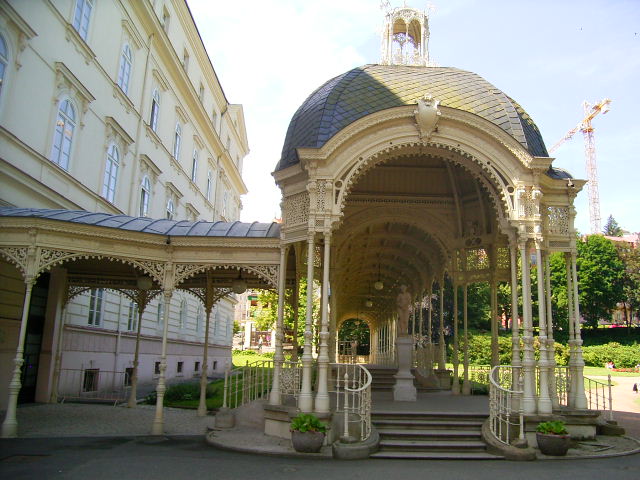The image portrays the front of a grand, multi-storied building, resembling a castle or a fancy hotel, beautifully set against a backdrop of a clear blue sky and green trees. The building itself features a cream-colored concrete facade adorned with rows of windows. To the left, a covered walkway with a blue tile roof and ornate scrolling designs connects to the front structure, enhancing its majestic appearance.

This front section boasts a long, arched roof supported by vertical rods, with artistic scrolling and intricate designs along its exterior. The walkway is open on all sides, allowing you to fully appreciate its architectural elegance. A staircase with curved handrails leads up to this arched area, where a statue of a human form, crafted from a material resembling concrete, stands on a pedestal. The overall aesthetic of the scene exudes a French regal charm, making it a striking and picturesque sight.